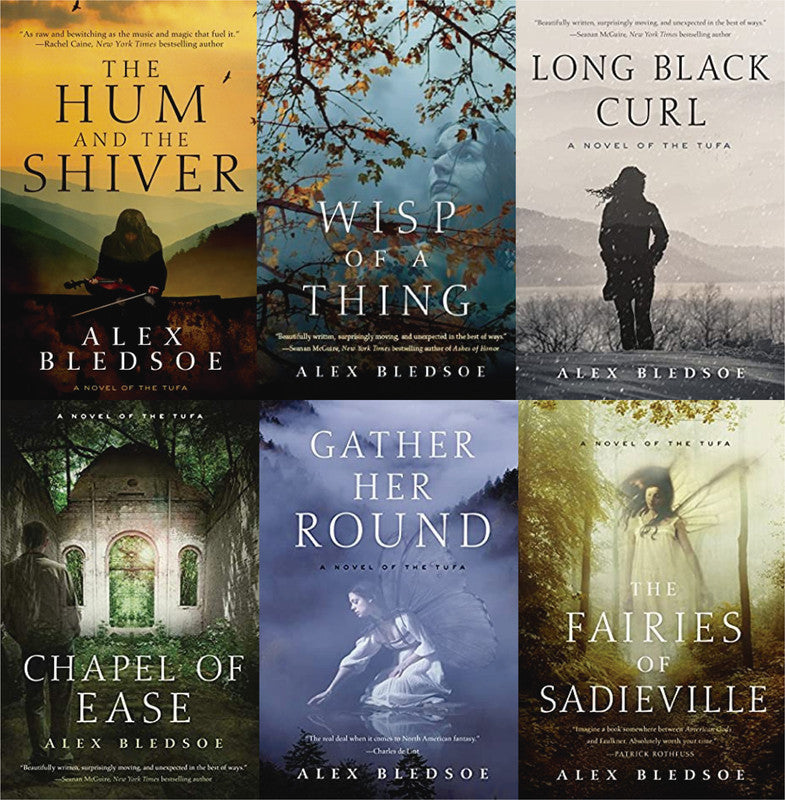This is an image of six ethereal and slightly melancholic book covers by the author Alex Bledsoe, each depicting elements of fairy tales and mythic themes. The first cover, titled "The Hum and the Shiver," features an orange-yellow background with a figure, possibly a man or woman, holding a violin, and is illustrated in white text. The second cover, "Wisp of a Thing," shows a woman gazing up at a sparsely leaved fall tree against a gray background, with the title in white text. The third cover, "Long Black Curl," portrays a woman walking in the snow with mountains and a lake in the background, also marked as "A Novel of the Tufa." The fourth cover, "Chapel of Ease," presents a man peering through a window of a derelict chapel in the woods. The fifth cover, "Gather Her Round," depicts a woman with fairy wings almost touching the surface of water. The sixth cover, "The Fairies of Sadieville," shows a young, ghost-like girl with fairy wings walking through the woods, her brown hair swept across her face. Each cover exudes a sense of magic intertwined with a hint of darkness or sadness, highlighting the enchanting themes characteristic of Alex Bledsoe's work.